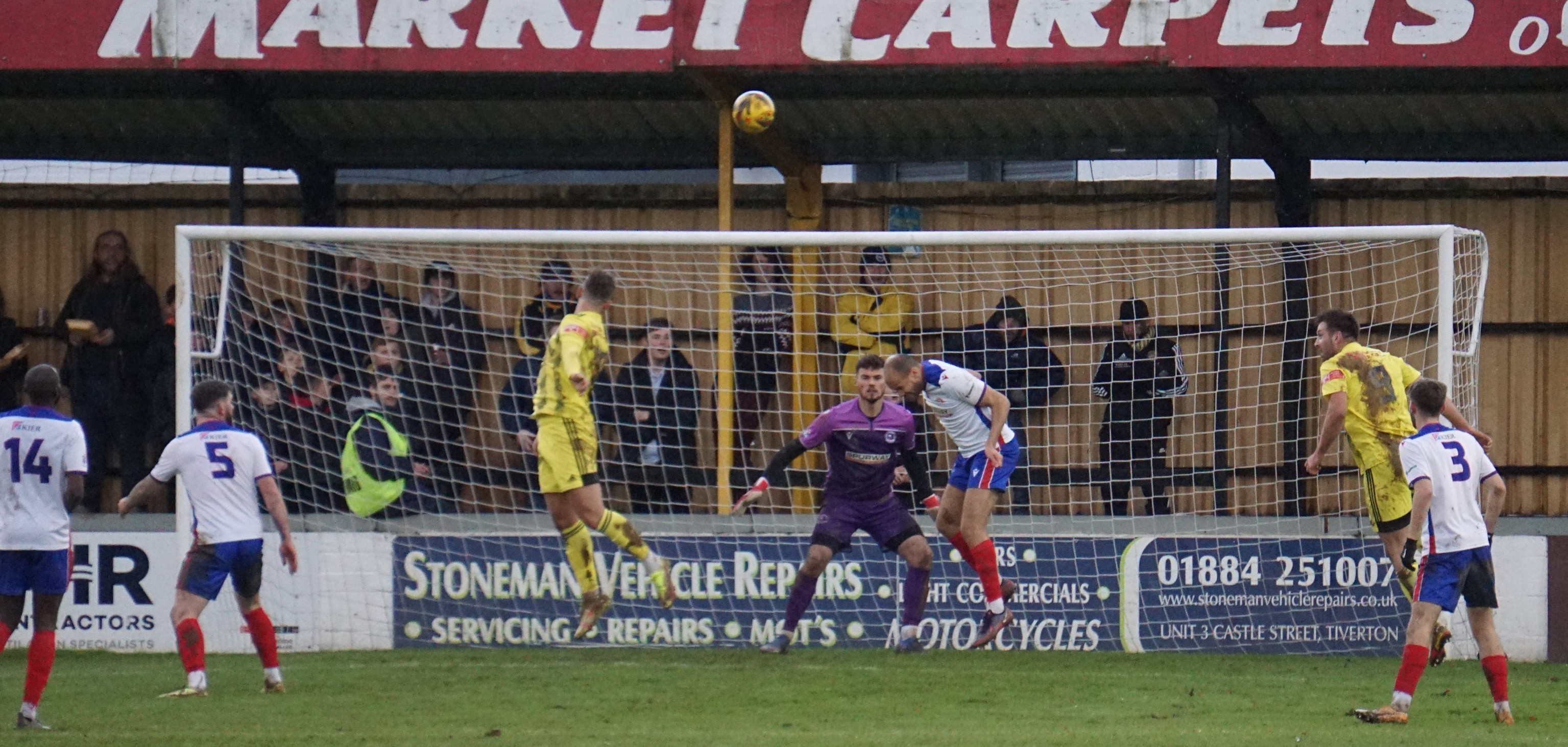In the middle of an intense soccer match, a player in a yellow uniform is captured mid-air executing a header. His body is perfectly angled for the move, indicating a high level of athleticism. The opposing team, clad in white shirts with blue shorts and red knee-high socks, includes two numbered players, 14 and 5, who are focused intently on the play. The yellow player's header directs the ball above the goal, leaving its trajectory uncertain. The goalie, dressed in a purple outfit with navy blue accents and navy blue socks, is poised with arms outstretched and knees bent, ready to intercept. To the right, more players in yellow and white uniforms watch the unfolding action. The green grass of the soccer field serves as the backdrop, framed by a goal that spans two-thirds of the picture's width. An audience in the background, along with visible banners, add to the competitive atmosphere of the scene.